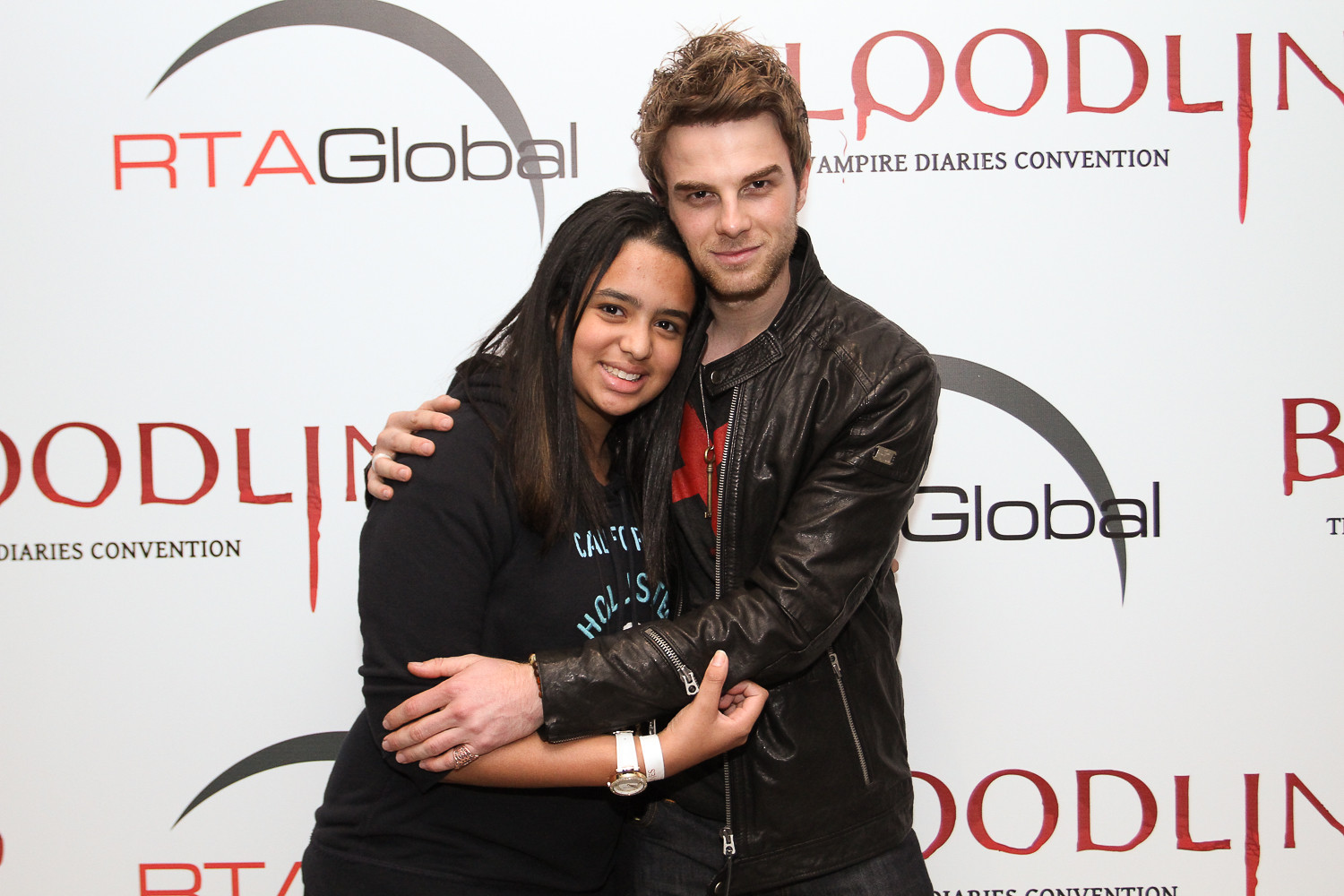In this fan photo taken at the Bloodline Vampire Diaries Convention, a young woman poses with a male star from the show against a promotional backdrop featuring the event's name alongside the RTA Global logo. The backdrop has the words "Bloodline Vampire Diaries Convention," with the design elements giving a nod to the vampire theme. The fan, with long, straight, dark hair and olive-toned skin, wears a black Hollister hoodie and accessorizes with a white bracelet and a white banded watch on her right arm. The actor, recognizable by his messy brown hair, five o'clock shadow, black leather jacket, and a black t-shirt featuring a red X, reciprocates her awkward hug. Both appear in their respective elements: the fan radiating excitement and admiration, and the actor graciously participating in the fan event.